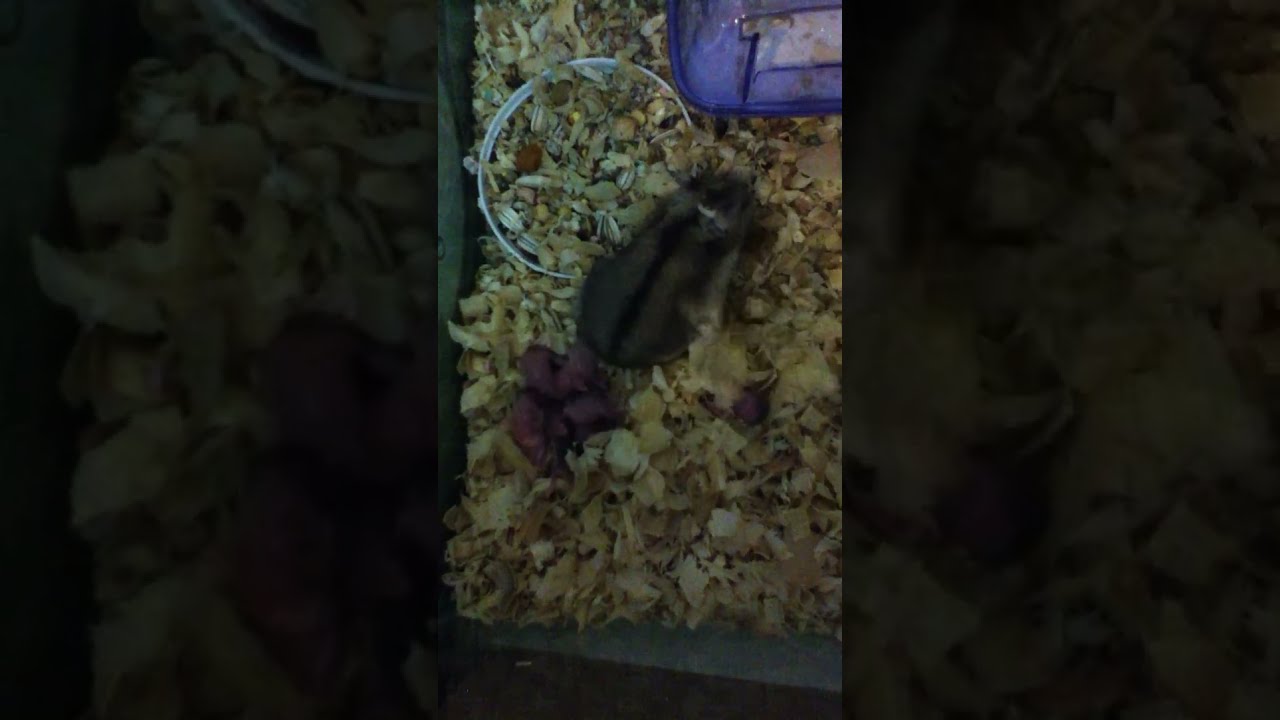This image is vertically divided into three sections, with the first and third sections completely covered in black. The middle section showcases a somewhat ambiguous scene dominated by what appears to be dried organic material or wood chips in various shades of light brown to brown. In this material, there are several small, reddish-brown and purple items that could be interpreted as either dry fruits or perhaps dried petals. A prominent circular white plate or wire bowl in the top left quadrant holds some of this material, partially embedded within it. On the far left and bottom edges, a wooden or dark brown-green box frames the contents. Additionally, there is a cluster of tiny, curled-up entities, pink and brown in color, that resemble either small animal babies or squiggly organic matter, with one isolated piece resting on the right side. The overall appearance is somewhat blurred, adding to the enigmatic nature of the scene.